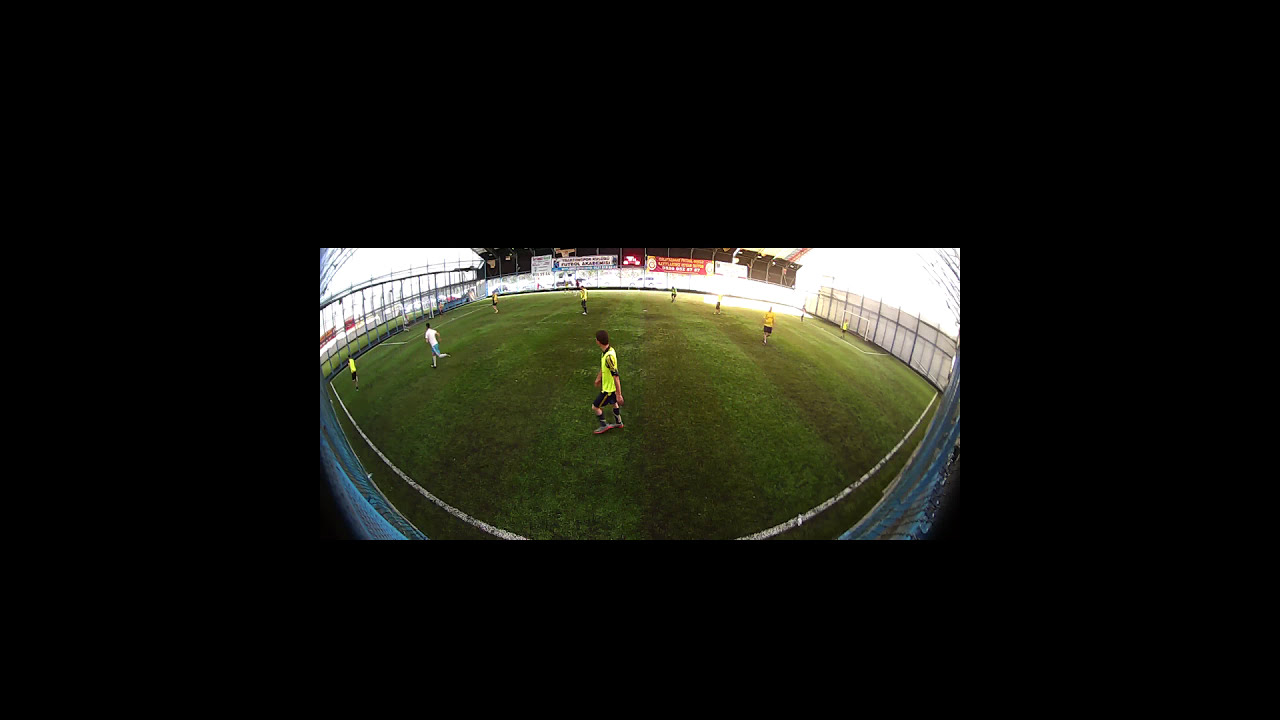The image captures an action-packed moment of a soccer game on a compact, enclosed field with vibrant green grass. Taken with a fisheye lens, the corners of the image curve dramatically inward, accentuating the smallness of the field. There are approximately twelve players on the field, divided into teams with distinct uniforms: one team in yellow jerseys paired with black shorts, and another in a mix of lime green and white jerseys. Both goals are visible, each with a goalie stationed alertly. Surrounding the field is a blue fence, adding a circular, enclosed feel to the setting. In the background, various red and white signs and banners hang above the fence, presumably displaying sponsors' names, though they are too distant to read. The sky above is a stark white, completing the scene.